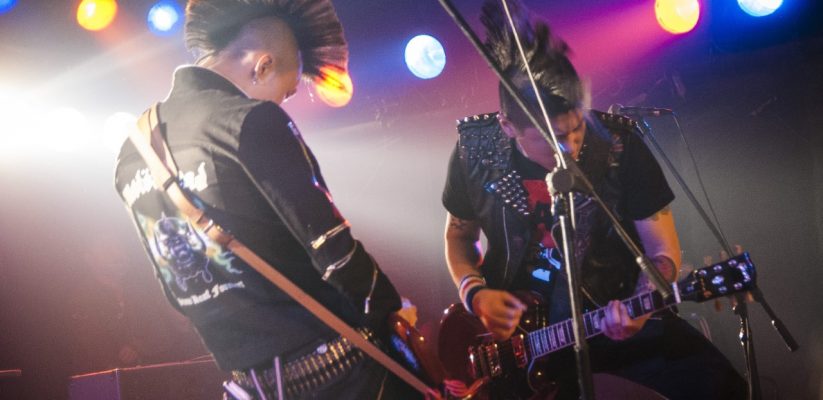This vibrant color photograph captures an electrifying moment at a concert venue featuring two band members, both jamming out intensely on their guitars. The musicians, each sporting tall, distinct mohawks, exude a rebellious rock aura. The man on the left, with partially shaved sides on his head, is clad in a long-sleeved black shirt adorned with silver bands and a design of a robot on the back. His counterpart on the right dons a black t-shirt with a front design, and a wristband in black, red, and white on his right hand, his hair scraggly on the sides. Both performers wear leather jackets, with the left one featuring numerous spikes and the right one zipped up. Enhancing their rockstar image, one man wears an earring and a belt buckle resembling ammunition. The left musician is leaning into his red guitar while colorful lights in yellow, blue, and white illuminate them from behind. Guitar straps cross their shoulders as they bend over their instruments, lost in the music. The stage setup includes visible microphones, and a subtle glimpse of the crowd can be seen beyond the stage, all contributing to the high-energy atmosphere of the concert.